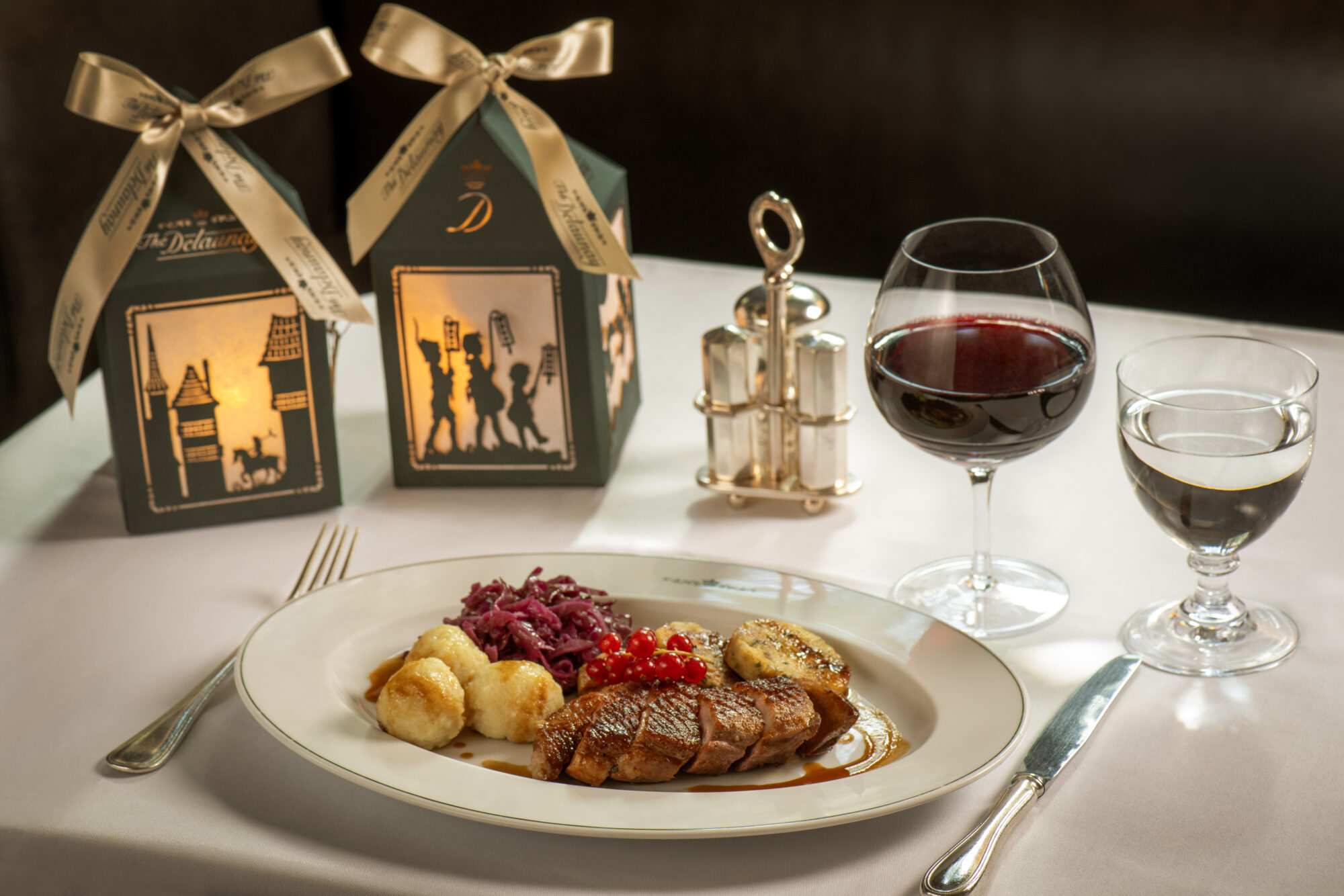The photograph captures an elegantly set table, likely prepared for a festive or special occasion, possibly a German or Austrian holiday event. The table features a pristine white tablecloth with a meticulously arranged place setting. At the center is an oval-shaped plate, its wide rim framing a beautifully presented dish that includes a succulent cut of meat, likely duck or pork, adorned with red currants. The plate also holds plantains or potato dumplings, and a portion of red cabbage or another pickled vegetable.

To the left of the plate lies a silver fork, while a matching knife rests to the right. Right behind the plate are a glass of rich red wine and a glass of water. Central to the table's arrangement is a stylish silver holder containing the salt and pepper shakers. Adding a decorative touch are two green favor boxes tied with gold bows, designed to look like ornate houses. These boxes feature intricate cutouts depicting scenes such as children holding lanterns and a person on horseback, possibly representing Saint Martin's Fest, a holiday known for its themes of light and generosity. The favor boxes glow softly, hinting at small lights within, contributing to the warm, sophisticated ambiance of the setting.